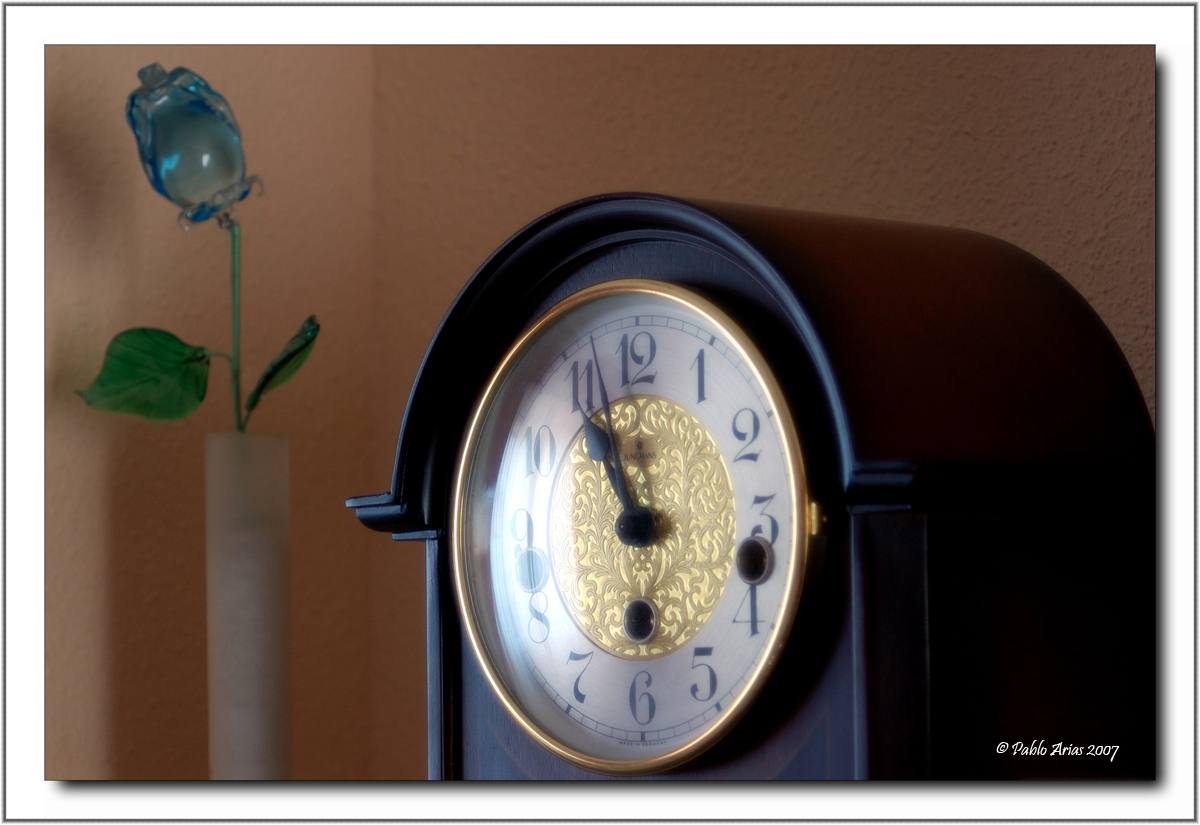A detailed and descriptive caption for the image could be:

"An artistic photograph capturing a vintage black clock positioned towards the right side of the frame. The clock features a round top and a gold face adorned with bold black numbers on a white backdrop, complemented by distinct black minute and hour hands. Set against a warm peach-colored wall, the scene is enhanced by a white vase with a greenish glass rose and accompanying greenery on the left. In the lower right corner, the image bears the text '© Pablo Area 2007,' denoting its artistic provenance. The composition collectively exudes a nostalgic and serene ambiance, blending classic timekeeping with delicate decor."